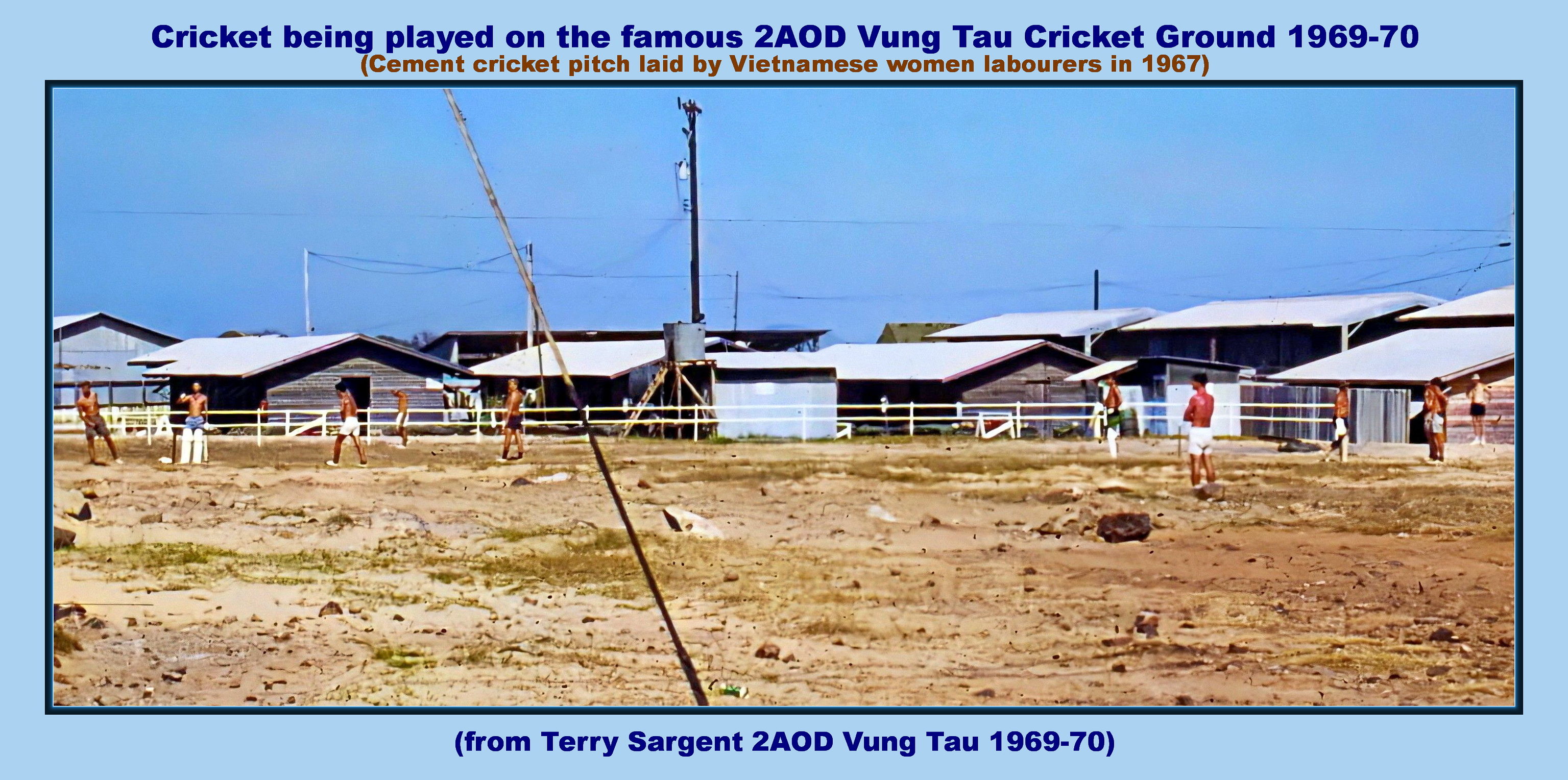This image features a postcard from Vietnam with a light blue border. The caption at the top in bold blue font reads, "Cricket being played on the famous 2AOD Vung Tau Cricket Ground, 1969-1970." Directly below this, in red font within parentheses, it mentions, "Cement cricket pitch laid by Vietnamese women laborers in 1967." The central rectangular photo showcases a desolate cricket field, primarily dirt with patches of grass and loose rocks. Several shirtless players, wearing various colored shorts, are visible playing cricket. The background includes multiple metal sheds with pitched roofs, resembling barracks, and a white fence separates the playing field from these buildings. The scene is captured on a bright, clear day with a vivid blue sky. At the bottom of the border, in parentheses and blue font, the caption credits the photo to "Terry Sargent, 2AOD Vung Tau, 1969-1970."